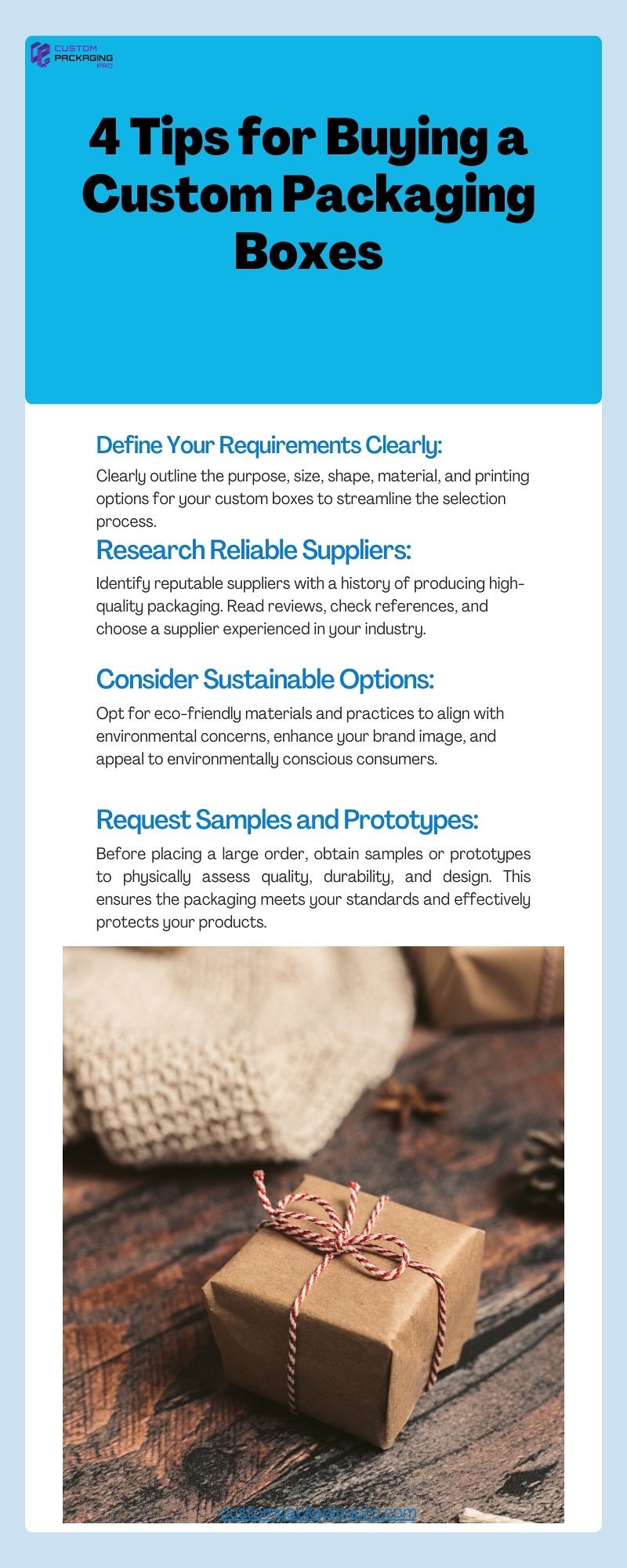The advertisement features a light blue background with the prominent black headline: "Four Tips for Buying Custom Packaging Boxes." Below this, in blue text, the tips are listed with black descriptions beneath each one. The tips include: "Define Your Requirements Clearly," "Research Reliable Suppliers," "Consider Sustainable Options," and "Request Samples and Prototypes." Underneath these tips, too small to read precisely, are further explanations of each point. The lower section of the ad shows a detailed shot of a brown paper package tied with decorative red and white twine, resting on an aged wooden table with a white blanket in the background.